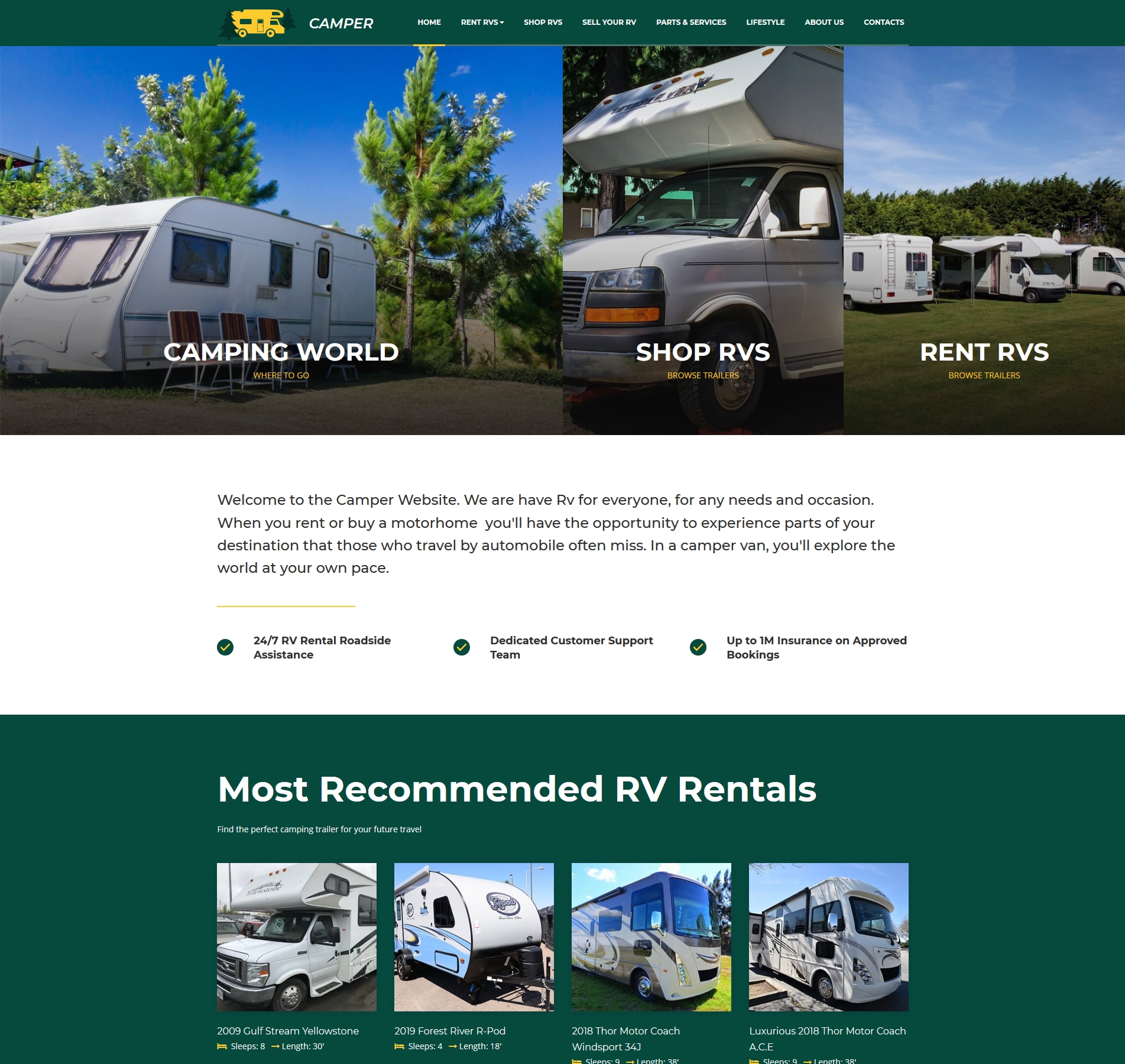The image features the homepage of the Camping World website. At the top left corner, there is a small yellow icon depicting a camper van, followed by the word "Camper." Below this, a horizontal menu bar with white background spans across the page, featuring categories from left to right: Home, Rent, Buy, Shop, Sell, Parts & Services, Lifestyle, About Us, and Contact Us. The text on these menus is quite small and might require closer inspection to read clearly.

Beneath the menu, there are three images arranged in a collage-like format. The first image shows a side view of a caravan with "Camping World" superimposed in white text. The second image features a camper van with the text "Shop RVs" overlaying the picture. The third image displays multiple camper vans parked in a field, with "Rent RVs" written on it.

In the center of the page, there's a predominantly white panel containing a welcoming paragraph at the top, introducing visitors to the Camping World website. This text is followed by three bullet points, each accompanied by a checkmark: "24/7 RV rental roadside assistance," "Dedicated customer support team," and "Up to $1 million insurance and approved bookings."

Underneath this central panel is a large, green section showcasing the "Most Recommended RV Models." This part of the site highlights four specific RV models, each accompanied by a detailed image, promoting the most rented vehicles available through Camping World.